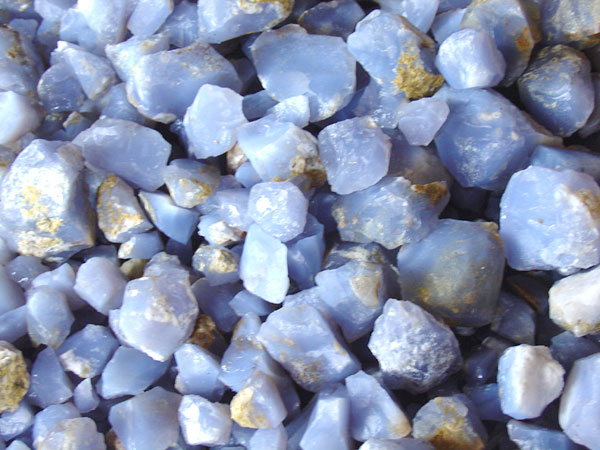In this detailed outdoor daytime photograph, the camera looks down onto a collection of light-colored pebbles and stones, arranged seemingly in a row, suggesting a beach setting or a rock collection. The stones range in size from about a quarter-inch to three-quarters of an inch and are irregularly shaped, with no perfect circles. Their color palette is predominantly a pale, chalky blue with milky white tones. Some stones feature splashes of yellowish-brown, adding a hard shell-like texture, while others reveal hints of agate or crystal characteristics, with minor reflections giving a shiny appearance. There are sporadic patches of moss or gold discoloration on the stones, contributing to their jagged, uneven texture, while some display smooth spots. Amongst the light blue stones are those with white or cream hues and occasional notes of greenish-yellow. Despite some claims of very pale or even purplish tones in parts of the stones, the consistent presence of white and brown, occasionally appearing golden, is notable. The absence of water emphasizes the earthy, raw aesthetic of the scene.